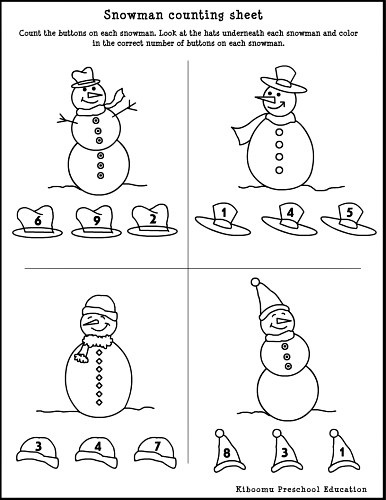This black and white image is a student worksheet titled "Snowman Counting Sheet" designed for preschool education, as indicated by the black text at the bottom right which reads "Kibumu Preschool Education." The worksheet features four uniquely drawn snowmen, each situated in a quadrant: top left, top right, bottom left, and bottom right. Each snowman is adorned with a different number of buttons and varying details, including some with arms and different types of hats, facial expressions, and directions they’re pointing.

The objective, clearly stated at the top of the worksheet, is for students to count the buttons on each snowman, select the corresponding hat beneath each snowman that displays the correct number, and then color in the correct number of buttons accordingly. 

The specific details are as follows:
- The snowman in the top left has six buttons, with options of hats beneath it marked with the numbers six, nine, and two.
- The snowman in the top right has four buttons, with options of hats marked one, four, and five.
- The snowman in the bottom left has seven buttons, with options of hats marked three, four, and seven.
- The snowman in the bottom right has three buttons, with options of hats marked eight, three, and one.

Notably, the two snowmen on the bottom have their eyes closed, and despite some lacking arms, all appear cheerful and are depicted with varied attire and expressions to enhance visual interest.